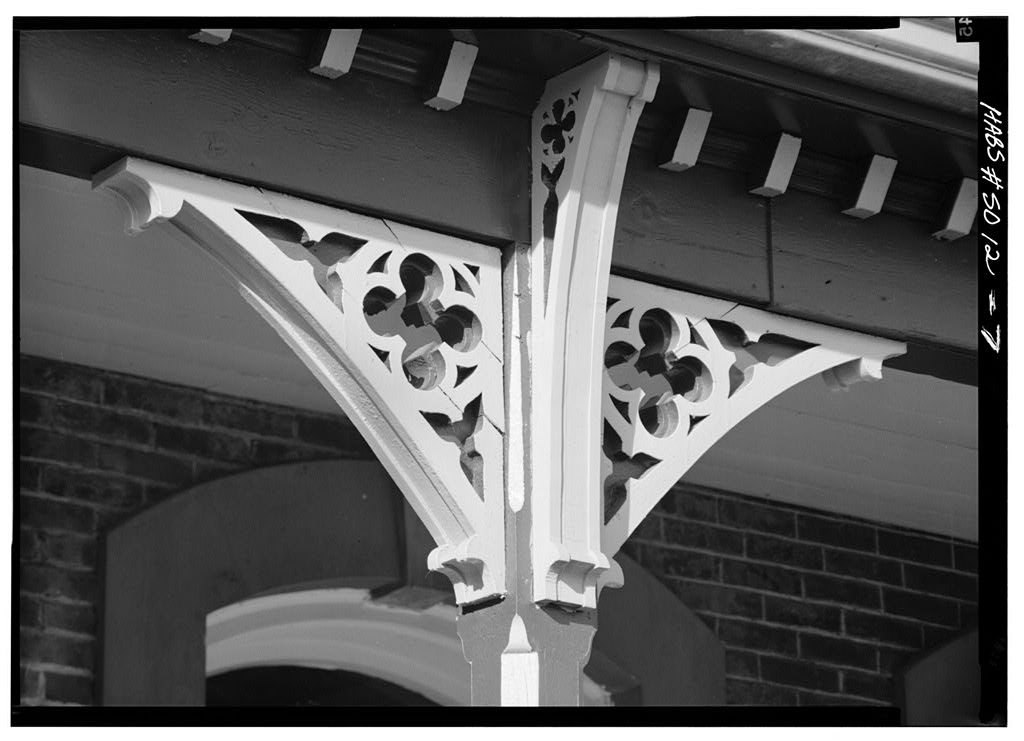The photograph depicts a detailed, black-and-white image of the exterior section of a building. Dominating the scene is the intricate eave of the rooftop, which is a grayish color with white accents. The eave features three-dimensional decorational pieces that include two triangular extensions, one pointing to the right and the other to the left, connecting to the roof via additional ornate elements. These white structures are hollowed out with various shapes, including a flower pattern, and exhibit a mix of curved semi-circles and angular 90-degree designs. 

Supporting the upper floor is a prominent white pillar in front of the eave. The photo cuts off part of the building, but you can glimpse the top of an archway below the eave. The building itself has a brick façade, with a distinct arch-top window partially visible behind the decorative elements. The overall craftsmanship and artistic details of the support post, along with the surrounding woodwork and brick wall, highlight the architectural beauty captured in this grayscale image.